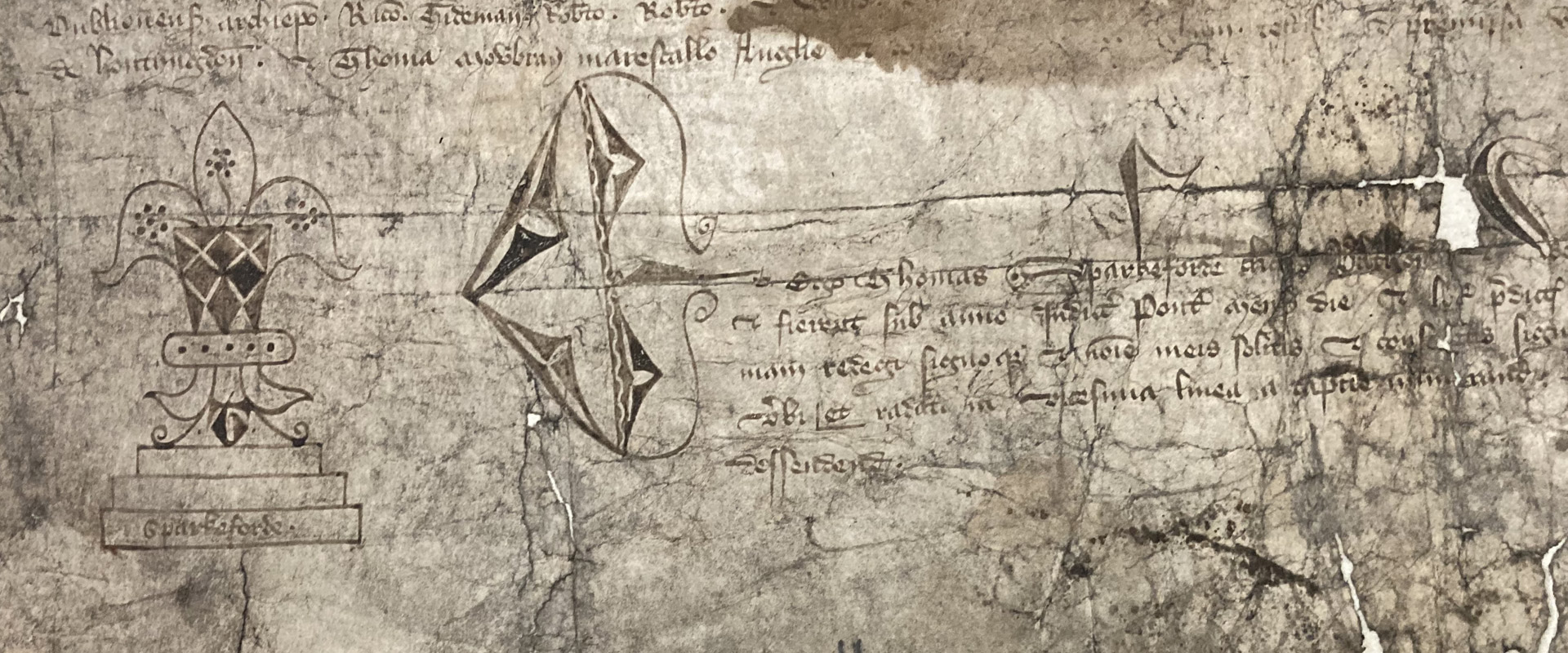The image depicts a piece of ancient, weathered paper, adorned with enigmatic, aged writing. The script, while unfamiliar, features characters that somewhat resemble those from old English texts, adding to its historical intrigue. Interspersed among the text are intricate symbols, the most prominent being on the left side - a design that appears to be a vase or a clover with three large leaves emerging from its base. This motif is echoed in several other spots across the paper. The document itself is significantly deteriorated, with noticeable wear and tear. A prominent hole on the upper right side reveals the surface beneath, highlighting the fragile and tattered state of the ancient paper.